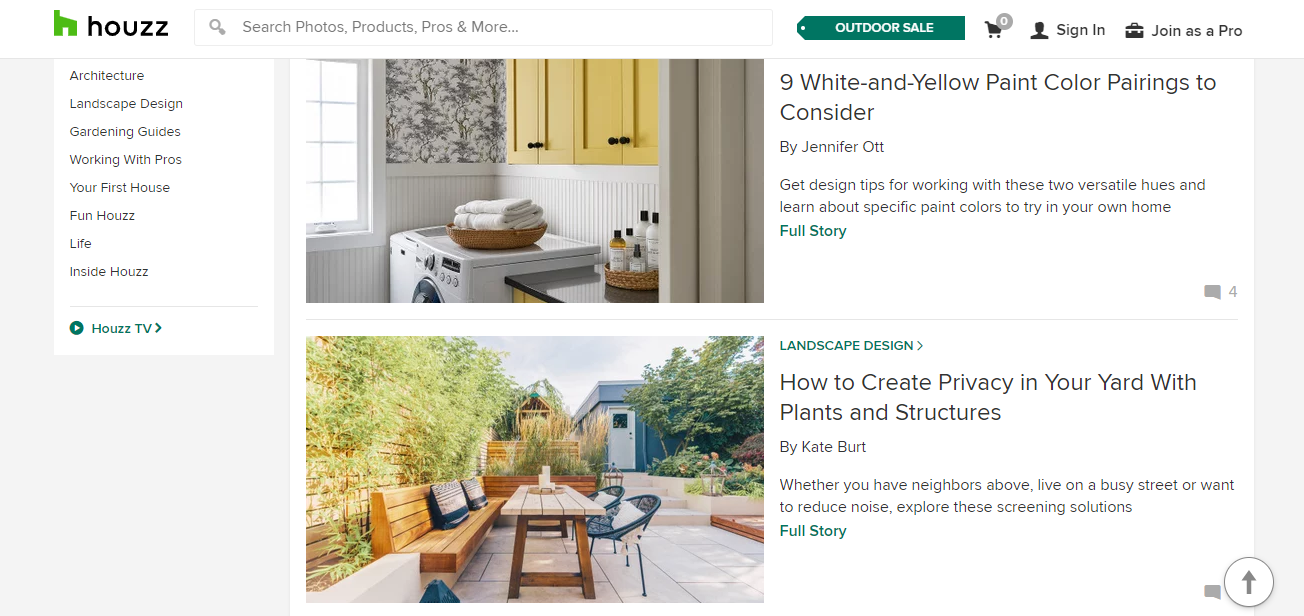The image is a screenshot from the website Houzz (H-O-U-Z-Z), detailing various sections users can explore. The top navigation bar features categories such as "Architecture," "Landscape Design," "Gardening Guides," "Working with Pros," "Your First House," "Fun House," "Life," and "Inside House." Towards the bottom right, there is an arrow leading to "Houzz TV."

On the right side of the screenshot, an image introduces an article titled "Nine White and Yellow-Pink Color Pairings to Consider." Below this, another section explains "How to Create Privacy in Your Yard with Plants and Structures."

At the top of the image, a picture showcases someone's laundry room, featuring yellow cupboards and predominantly white shelving. The bottom portion displays a serene backyard view, adding a touch of outdoor appeal to the page.